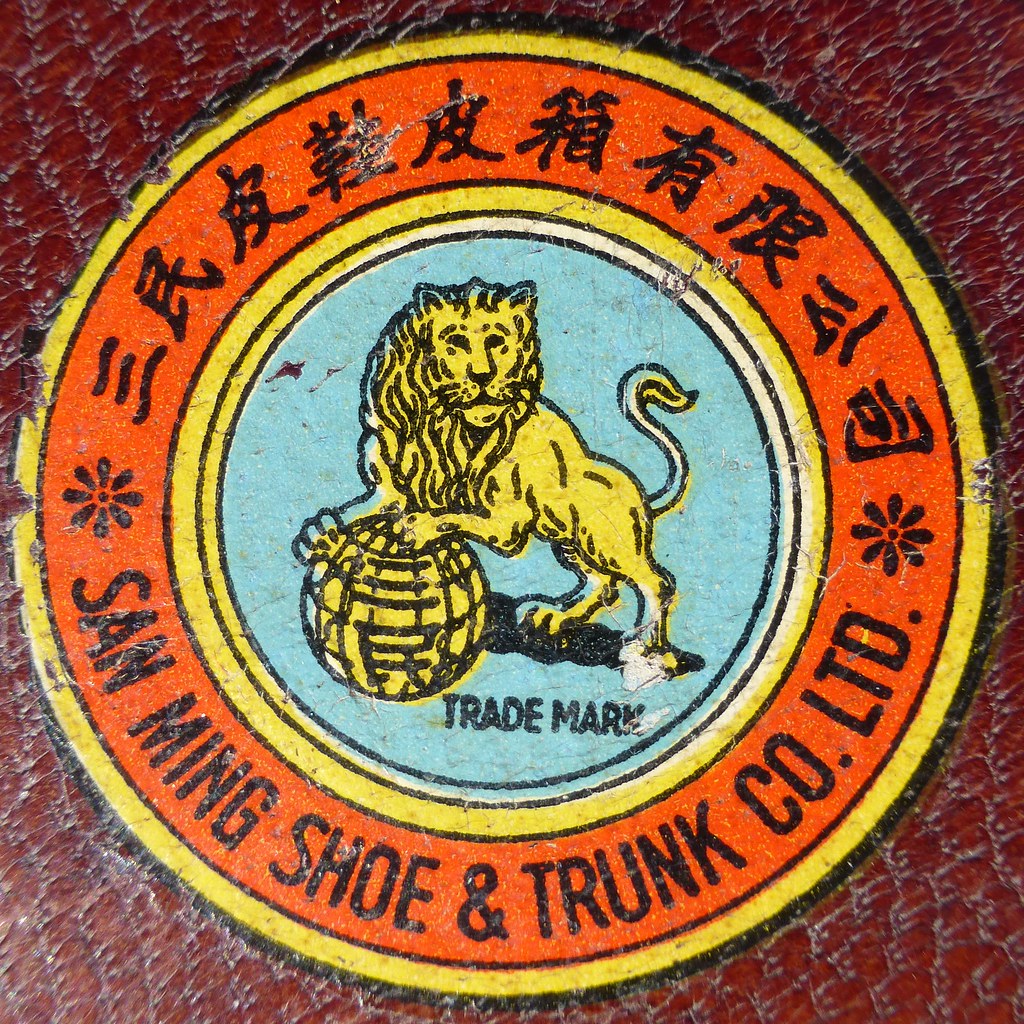The image showcases an old, circular company logo, possibly on a leather suitcase, with an amber-colored background featuring white streaks and evident wear and tear. The logo itself has a distinct multi-ring structure. The outermost ring is black, followed by a yellow ring, then a thick orange ring inscribed with black characters in an Asian language at the top and "San Ming Shu and Trung Ko period, LTD" at the bottom. Inside this orange ring lies another yellow ring encircling a central area with a light blue background. This central section features a detailed drawing of a lion standing on his back legs, facing left but with its head turned forward. The lion, primarily yellow with occasional blue spots where the color is missing, appears animated and reminiscent of the lion from "The Wizard of Oz." The lion holds a globe, which is intricately painted yellow with black lines, under its front paws, and the word "trademark" is inscribed nearby. The logo's worn condition, with scratches and a notable white mark obscuring the lion's bottom back foot, suggests it is from an earlier era.